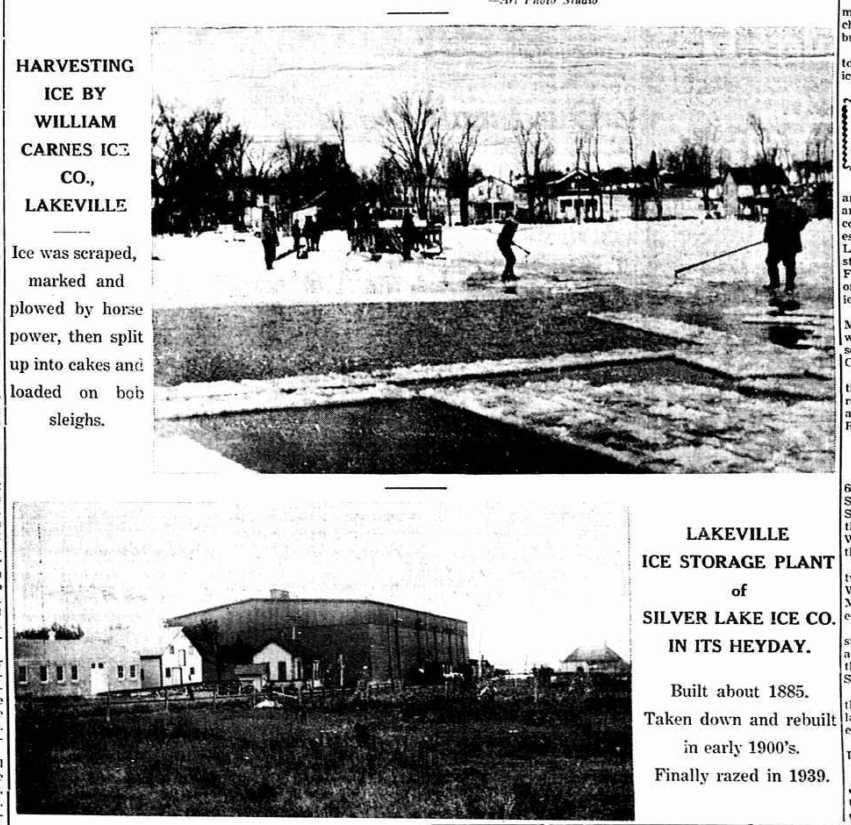The image appears to be a black and white reproduction reminiscent of a magazine or newspaper, possibly copied through a Xerox machine, which has resulted in a somewhat poor quality. It features two distinct photographs accompanied by explanatory text on the left. The first photograph details the ice harvesting process carried out by the William Carnes Ice Company of Lakeville. The text explains that the ice was scraped, marked, and plowed by horsepower before being split into cakes and loaded onto bobsleds. In this image, several people are seen working amidst what appears to be a wintery landscape with trees and homes faintly visible in the background. The second photograph, situated below the first, depicts the Lakeville Ice Storage Plant managed by the Silver Lake Ice Company. The scene includes a barn-like structure surrounded by a fence, with some overexposed grass in the foreground. According to the accompanying text, this plant was originally built in 1885, was taken down and rebuilt in the early 1900s, and was finally razed in 1939. Both images and text are in black and white, consistent with the newspaper-like aesthetic.